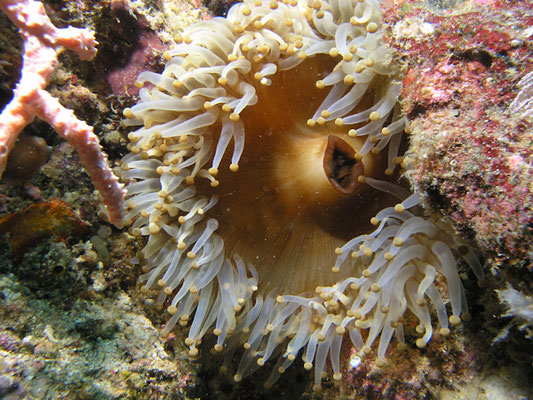The image depicts an underwater scene, possibly taken in the ocean or an aquarium, featuring a central sea anemone surrounded by rocks and coral. The anemone, which has an off-brown base, is adorned with numerous white, stringy tentacles, each ending in a distinctive yellow bulb. At the center of the anemone, there's a dark yellow cavity resembling a mouth. The surrounding environment includes pink coral with rough, spiky textures and areas of brown and white rocky formations. Algae might be present on some of the rocks on the right side. Flecks of sediment float in the water, adding to the authentic underwater ambiance. The lighting highlights the vivid colors and varied textures, bringing clarity to the intricate details of this marine scene.